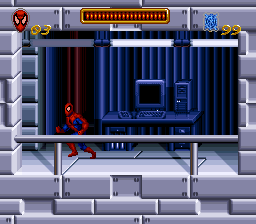In this color image, reminiscent of older video games with graphics akin to classic Sega style, we see a screenshot from a Spider-Man game. The scene shows Spider-Man, donned in his iconic red and blue costume with white, black-outlined eyes, positioned in a gray stone industrial building. He appears to be walking away from a blue desk with a computer, having just passed it. The background also features an open doorway or balcony with a view of an exterior brick wall. 

The game interface includes a red icon of Spider-Man's head in the top left corner indicating three lives remaining with "03" next to it. In the top right corner, there is a blue web icon showing that he has 99 web slingers left. Additionally, a red health bar at the top of the screen suggests that Spider-Man currently has full health. The overall depiction conveys an older, less advanced graphical style, adding a nostalgic charm to the gaming experience.